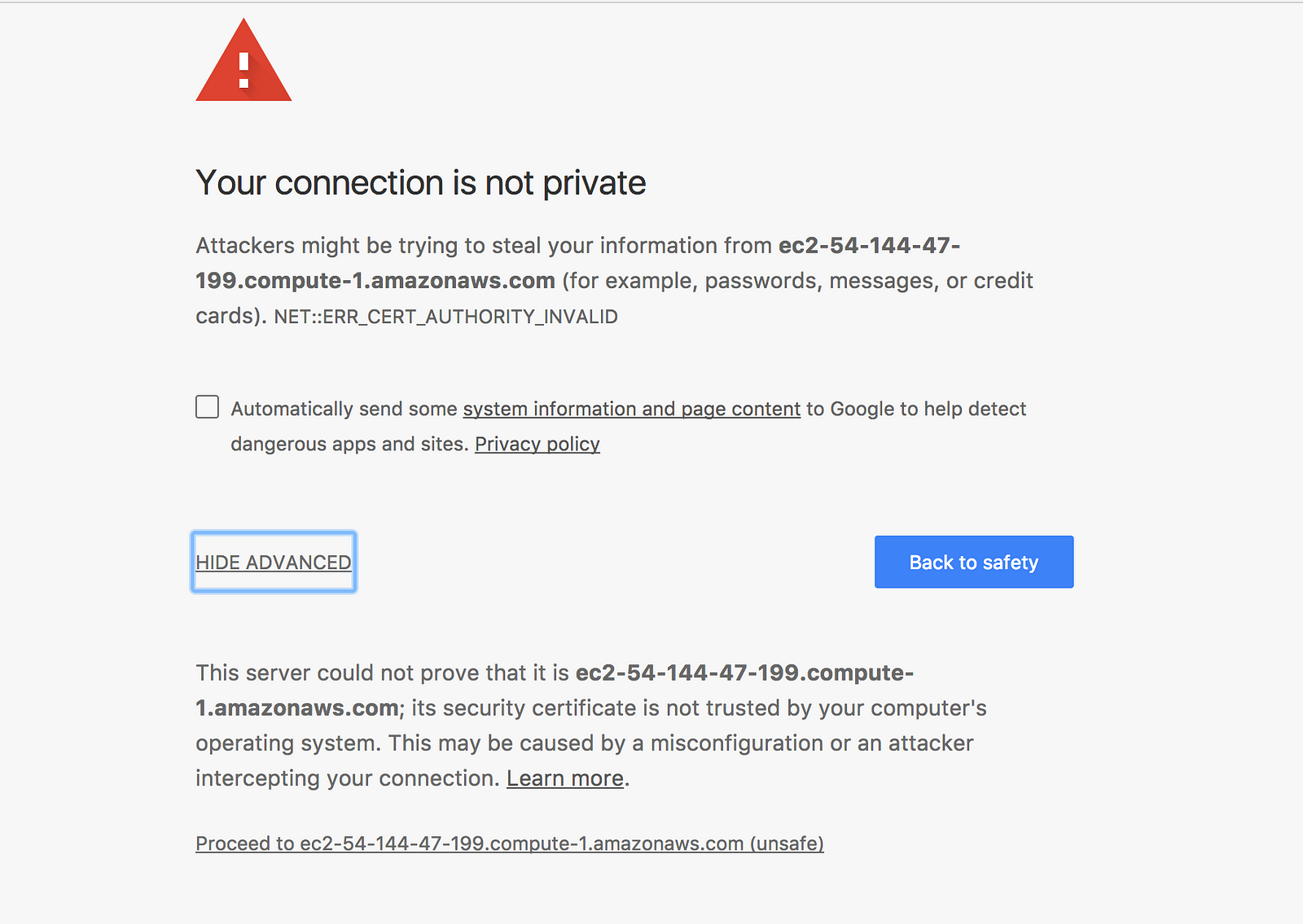The screenshot depicts a Chrome browser warning page that alerts users that their connection is not private. At the top, a red triangle with a white exclamation mark signifies a critical issue. The background is a plain, off-white grayish color, typical of Chrome's warning pages.

The primary message warns, "Your connection is not private." The detailed description below reads, "Attackers might be trying to steal your information from ec-54-144-47-199.compute-1.amazonaws.com," citing examples such as passwords, messages, or credit card details. The error explanation notes that the certificate authority is invalid.

An unchecked checkbox is visible, offering users the option to automatically send system information and page content to Google to help detect dangerous apps and sites, with a link to the privacy policy. The "Hide advanced" option is currently showing advanced information, explaining that the server cannot prove it is the site stated and that its security certificate is not trusted by the computer's operating system. This issue could be due to misconfiguration or an attacker intercepting the connection. 

To the right, a blue rectangular button labeled "BACK TO SAFETY" in white text is prominently displayed, urging users to return to a safer page. Additionally, there's another link providing more information and an option to proceed to the website despite the risks, marked as unsafe in parentheses.